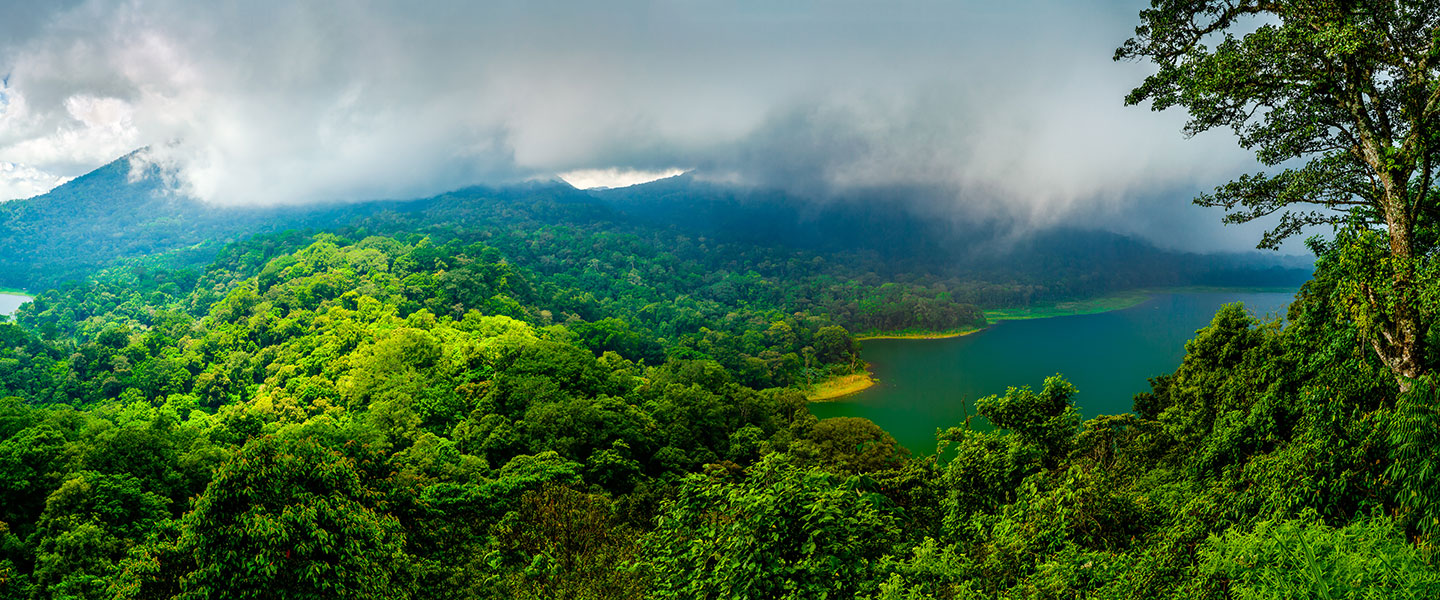This captivating photograph appears to capture a lush section of the Amazon rainforest, potentially situated in Brazil. The scene is dominated by dense, verdant greenery, with a land formation densely covered in trees stretching across the middle of a large body of water, possibly a lake or river. This natural formation gives the impression of an island surrounded by water on both sides. In the background, low-hanging, thick clouds obscure what could either be large mountains or dormant volcanoes, adding an air of mystery and beauty to the landscape. The absence of human activity enhances the tranquility, presenting an idyllic and serene snapshot of nature on a cool, cloudy day.